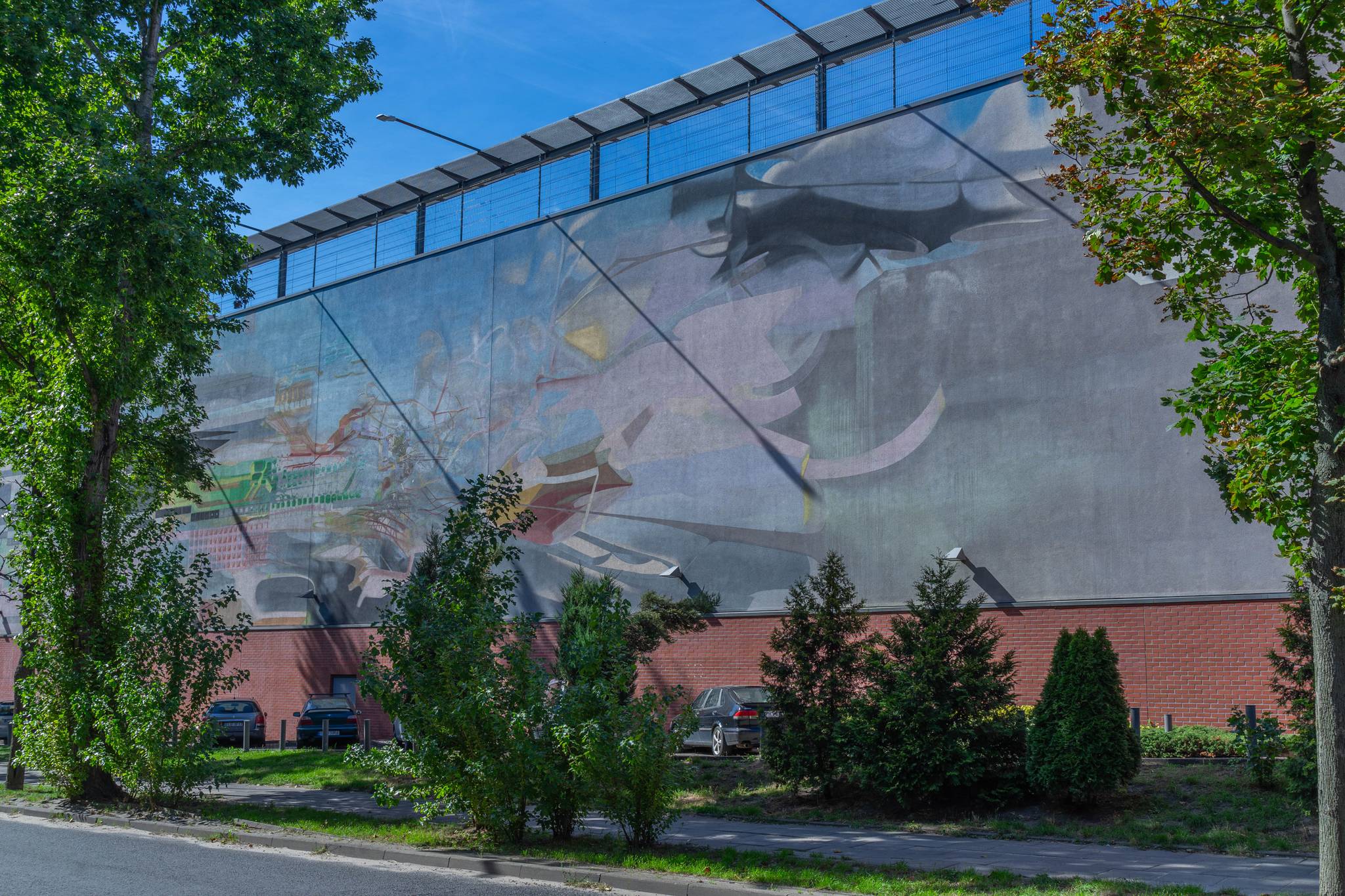This color photograph captures a large mural on the side of a building, meticulously detailed with a combination of abstract blue and green hues, along with various black and light gray shapes. The mural, evoking images of a water scenario, perhaps akin to an artistic representation of fish swimming, is prominently featured on a wall composed of a lower section of red brick topped with plain concrete. Above the mural, a strip of windows reflects the bright blue sky, with lights projecting from the rooftop to illuminate the artwork. The foreground showcases an asphalt road with a curb, a sidewalk, and three green trees lining the roadway, accompanied by small shrubs. In front of the building, a parking lot accommodates several vehicles facing the mural. The overall setting suggests a serene and inviting atmosphere, possibly reminiscent of a park or a recreational area.